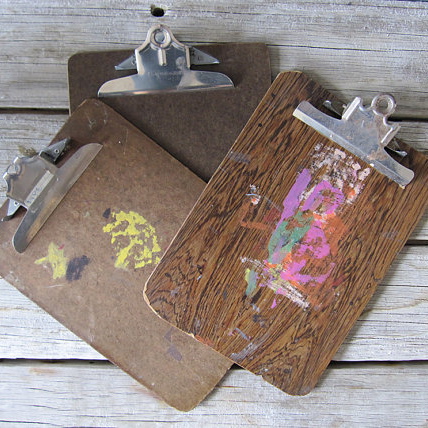The image features a weathered, white-washed wooden background, showing visible wood grain and patches of brown and gray. Three brown clipboards with silver clasps are arranged on top of each other in varying angles. The topmost clipboard, leaning towards the right, is marbled brown with several colorful paint stains in white, purple, orange, green, pink, and gray. The middle clipboard, positioned with a slight left orientation, is a lighter brown with remnants of yellow and black paint, suggesting a partially peeled yellow sticker. The bottom clipboard, barely visible, is a darker brown and largely paint-free. The entire scene is viewed from above, highlighting the rustic aesthetic of both the clipboards and the table.